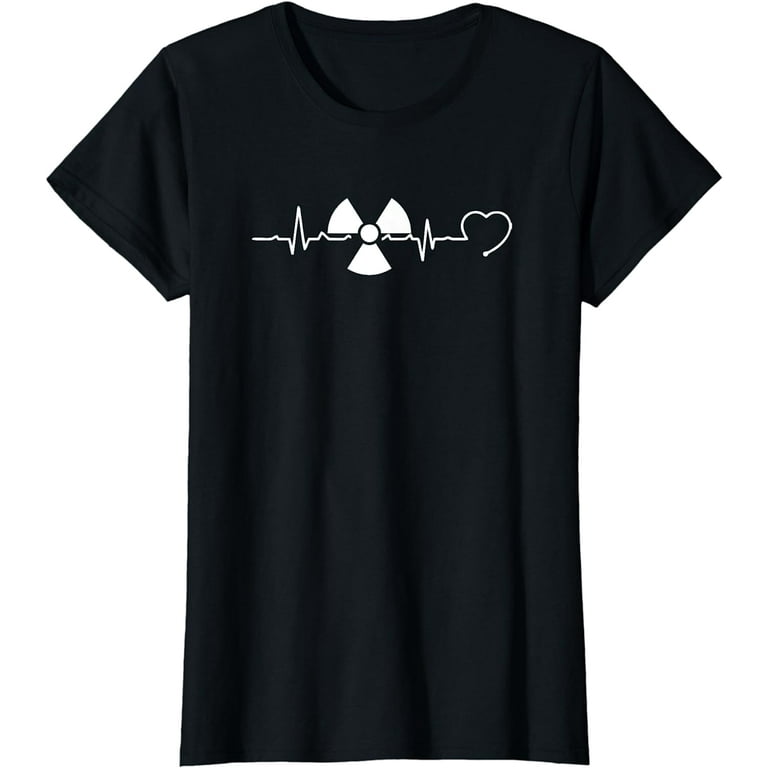The image features a plain black t-shirt with short sleeves, set against a white background. The main design on the front of the t-shirt consists of a series of intricate white lines. Central to the design is a symbol that closely resembles a radiation symbol, characterized by a white circle with three equally-sized sections radiating from it, resembling blades or fans. This symbol is positioned at the middle of the chest area. Behind the radiation symbol is a pattern that mimics the appearance of an EKG heartbeat line, which meanders across the shirt. To the far right of the pattern, the line transitions into an unfinished heart shape, providing a subtle yet distinct touch to the overall design. The entire pattern is rendered in white, creating a stark contrast against the black fabric of the t-shirt.